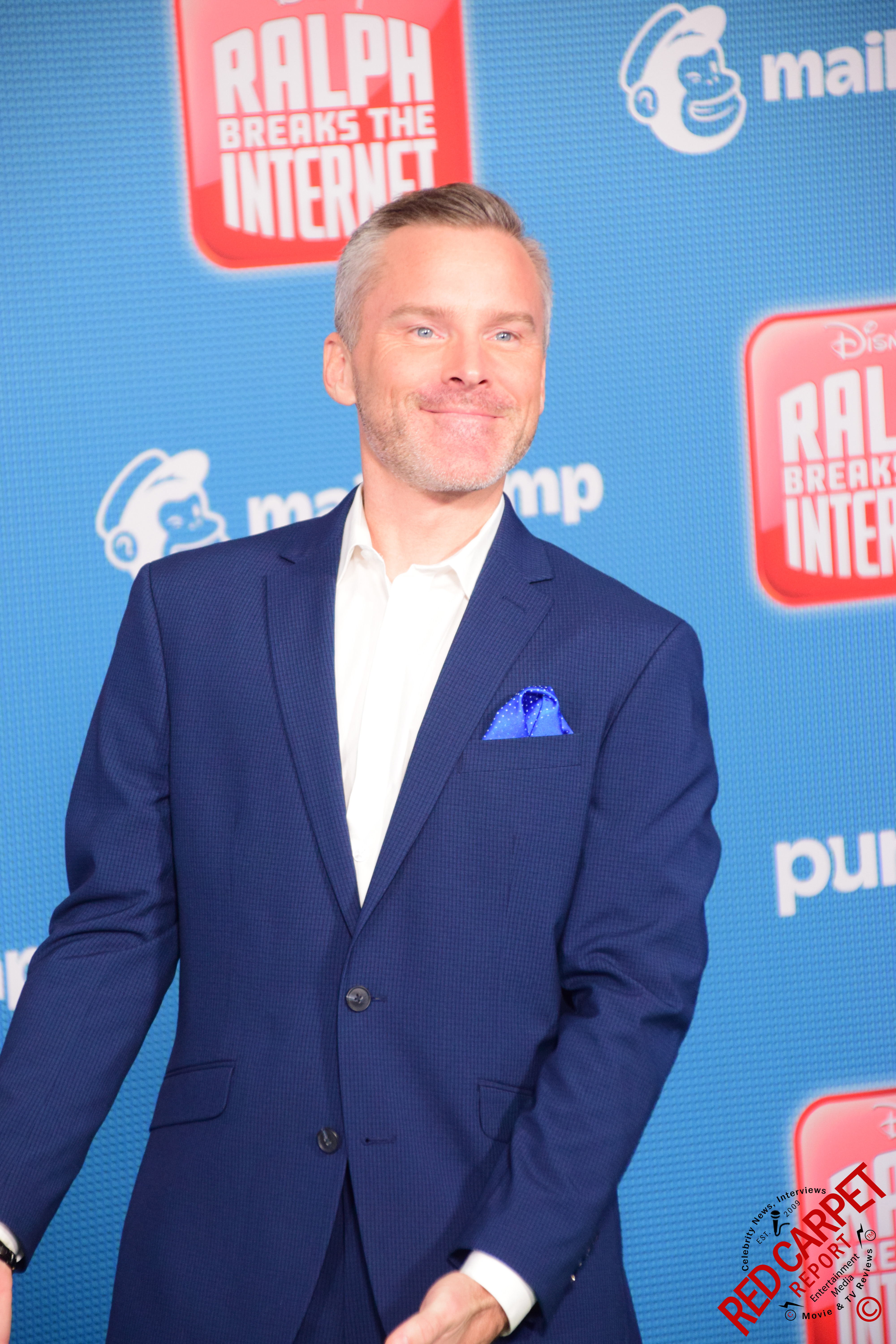In this indoor image, a man dressed in a dark blue suit stands prominently at the center, exuding a formal and polished presence. Behind him, a backdrop adorned with various posters and signage sets the scene. Among these, a particular poster catches the eye, featuring an image of a monkey with the caption "Male Chimp." Adjacent to this is the recognizable logo for "Disney's Ralph Breaks the Internet." At the bottom of the backdrop, the mark of "Red Carpet Report" is visible, indicating an event coverage. The color palette of the image includes dark blue, blue, white, gray, tan, red, and white, adding vibrancy and dimension to the scene. The man’s position and the detailed backdrop suggest the photo was taken during a notable event, possibly a movie release or premiere.